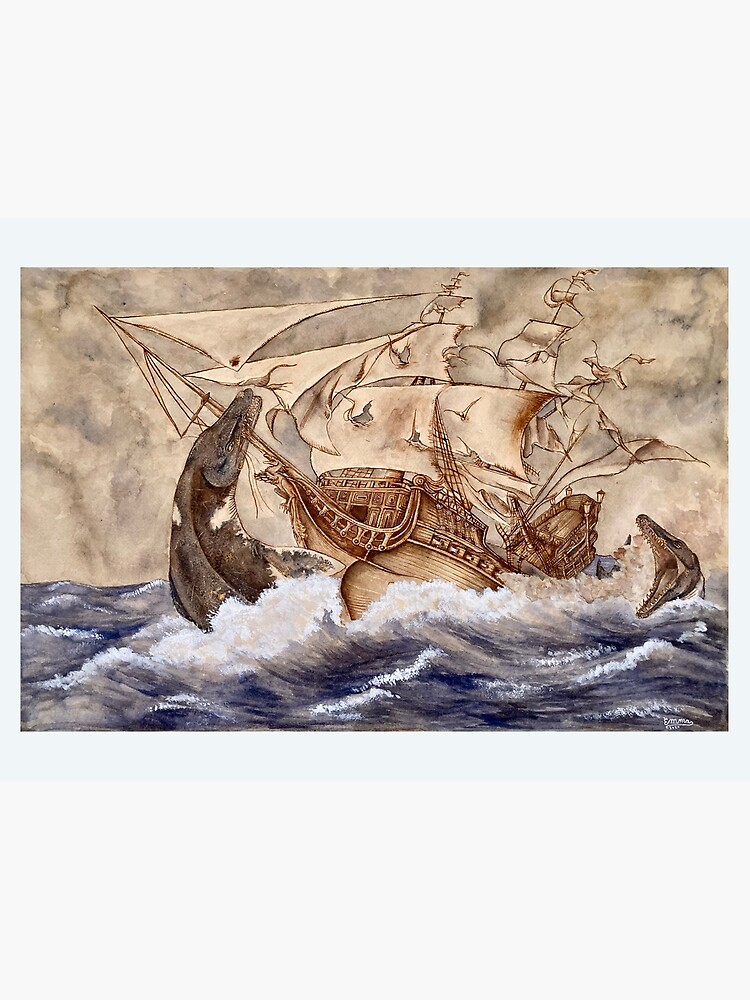The painting depicts an old English sailing vessel battling two massive, unrecognizable sea creatures in a turbulent, overcast ocean. The canvas is dominated by muted tones of brown and gray with accents of cream and gold, giving it a vintage appearance. The choppy sea, rendered in light blue and gray with white foaming crests, suggests a storm or the turmoil caused by the creatures. One sea creature, reminiscent of aquatic dinosaurs like Ichthyodon, with a long neck and pointed nose, bites the ship's prow, while the other menacingly roars with its mouth open towards the ship's starboard side, which is already cracked in half. The ship, tan with tattered white sails, appears to be lifted out of the water by one creature, suggesting a fierce attack, with the sky above heavy with ominous clouds. The creatures, brownish-gray with white spots under their necks, add a menacing, surreal quality to the dramatic scene.